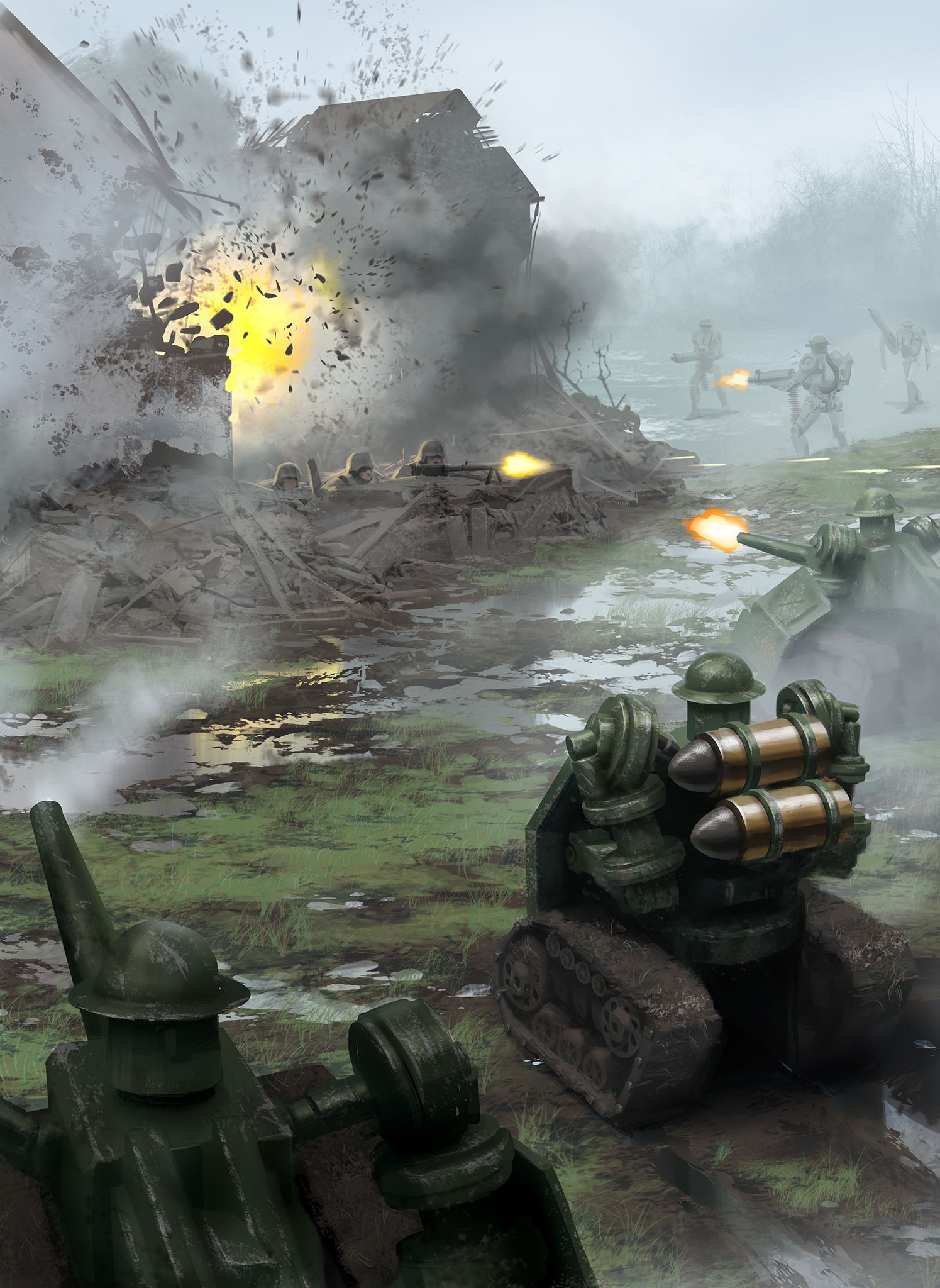The illustration portrays an intense wartime scenario set in a muddy, tattered battlefield with scattered puddles and debris. Central to the scene, a structure is under heavy assault from various war instruments, including oddly shaped, perhaps fictional tanks—some with exaggeratedly large ammunition strapped to their backs. These small tanks move through the chaotic, smoky landscape, with three visible tanks, one of which is partially obscured in the background. Soldiers on both sides are engaged in fierce combat; those defending the structure return fire, while attackers advance, their weapons discharging visible muzzle flashes. The air is thick with white and black smoke and mist, further dramatized by an explosion within the structure, which sends debris flying. The background reveals trees shrouded in the pervasive fog of war.